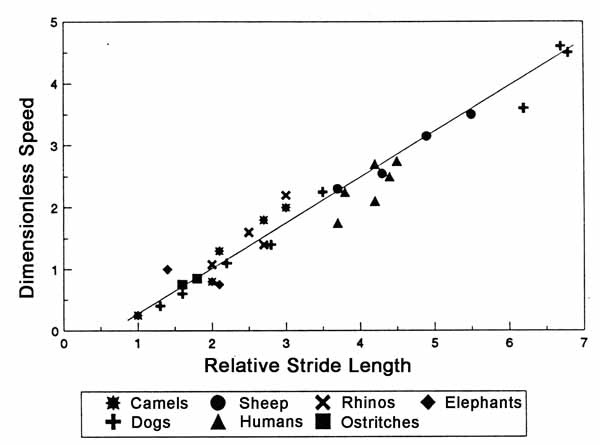This black and white scientific graph illustrates the relationship between dimensionless speed and relative stride length. The y-axis, labeled "dimensionless speed," ranges from 0 to 5, while the x-axis, labeled "relative stride length," ranges from 0 to 7. A thin black line diagonally traverses the graph from the bottom left to the top right corner, showcasing various data points represented by different black shapes such as X's, squares, circles, triangles, plus signs, diamonds, and asterisks. The key beneath the graph identifies these shapes: asterisks for camels, plus signs for dogs, circles for sheep, triangles for humans, X's for rhinos, squares for ostriches, and diamonds for elephants.